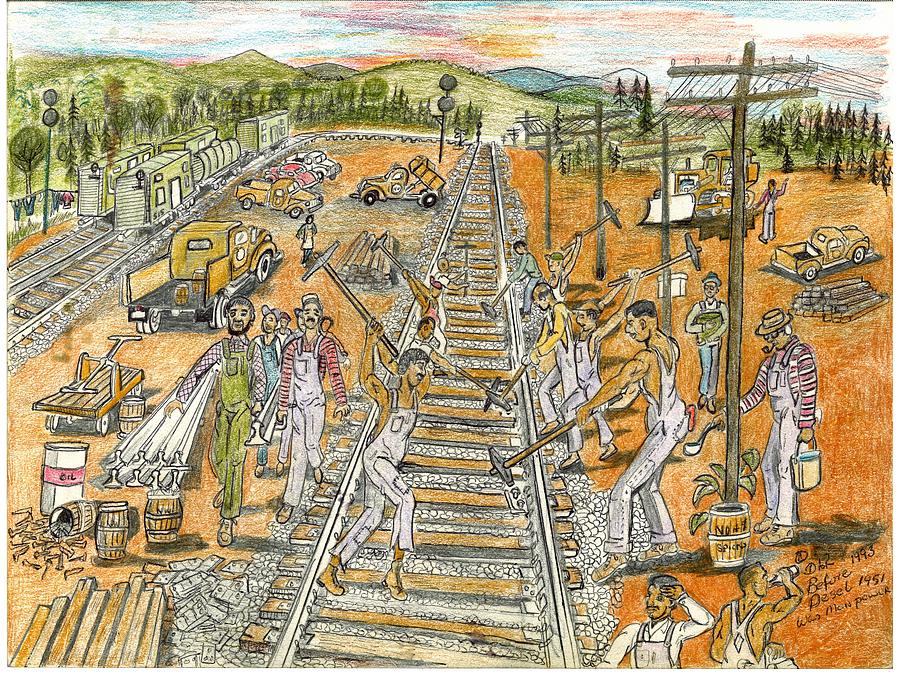This detailed colored pencil drawing vividly depicts a bustling scene of railroad workers laboring diligently on railway tracks that stretch vertically into the background. The central focus is the railroad made of brown wood slats and metal, flanked by shirtless men in white overalls wielding axes and hammers, engrossed in their efforts to construct the track. To the left, more workers in overalls walk along and carry pieces of steel, possibly for track construction. Among them, various colorful trucks—orange, white, and red—and green train carts are visible, with additional tracks running parallel. In the top left, a group of six workers in white overalls walk toward the viewer.

Dominating the background, green hills roll gently under a dynamic sky, awash with hues of red, blue, orange, and pink, applied in visible pencil strokes. To the right, a patch of brown ground features a row of electrical wire poles extending into the distance. Nestled amidst trees, a yellow old-timey truck and a bulldozer are stationed near a stack of wooden logs. Near this machinery, a worker in a red shirt and beige slacks stands by an orange truck, while another worker in white overalls drinks from a bottle, capturing a moment of respite.

The bottom right of the image bears the artist's signature, followed by the inscriptions "1993, before diesel, 1951, was manpower," marking a poignant reflection on the era depicted.